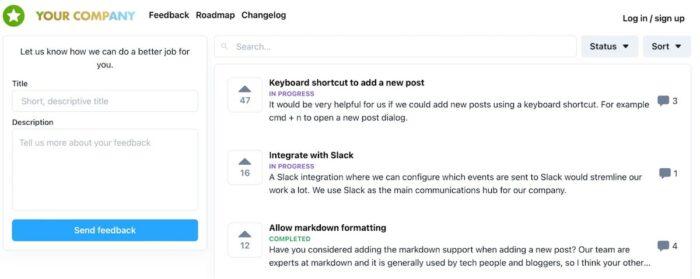The image is a screenshot showcasing a user feedback and feature request platform for a company. On the left side, there is a green circle with a white star inside it. Adjacent to this, in a gradient text that transitions from green to gray, the company name "Your Company" is displayed. 

Ahead in the header, there are navigation options in black text that read "Feedback," "Roadmap," and "Changelog." On the right-hand side of this header, there are options to "Login" or "Sign Up."

Below the header, on the left side, there is a prompt that says, "Let us know how we can do a better job for you." Beneath this prompt, a section is provided where users can write a short description of their feedback. An accompanying textbox allows detailed feedback input.

At the bottom of this section, a blue rectangle button with white text reads "Send Feedback." 

To the right side of the main content area, there is a search bar labeled "Search" along with options to filter feedback by "Status" or "New." Additionally, there is support for keyboard shortcuts and options to post comments.

Three feature suggestions are listed: 
1. "Integrated with Slack" with three comments.
2. "Allow Markdown formatting" with four comments.

The layout is clean and functional, focusing on user interaction and feedback submission.